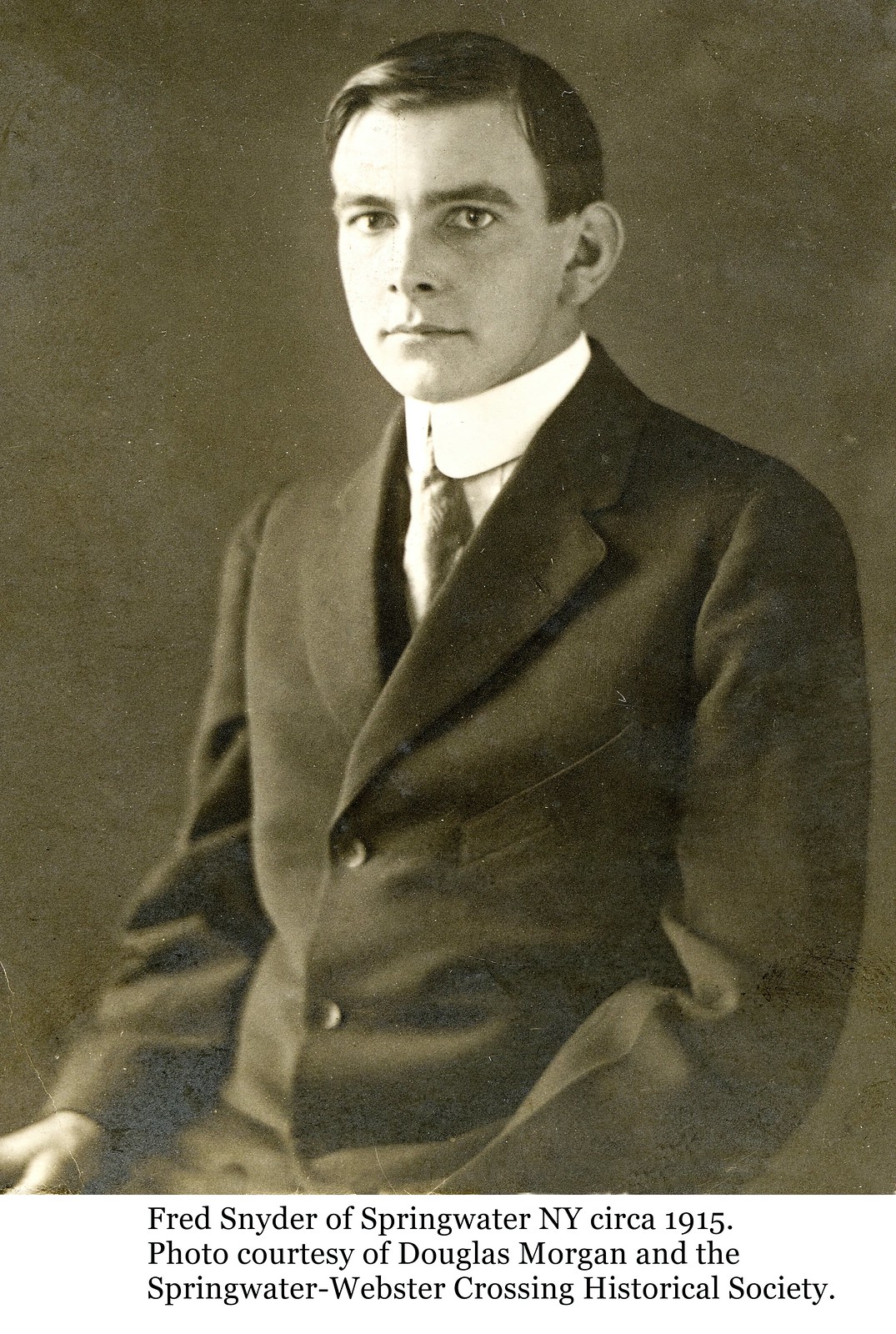This is a detailed black-and-white photograph, approximately 108 years old, of a man named Fred Snyder from Springwater, New York, circa 1915. In this solemn portrait, Fred is dressed in a dark suit paired with a light-colored shirt and a tie. He has short, straight hair, dark eyebrows, and open eyes, giving him a composed but serious expression. Sitting down, Fred rests his right hand on his right leg and his left hand on his left leg, suggesting a formal pose typical of early 20th-century photography. The bottom of the photograph contains an inscription in dark print that reads, "Fred Snyder, Springwater, New York, circa 1915, photo courtesy of Douglas Morgan and the Springwater-Webster Crossing Historical Society".